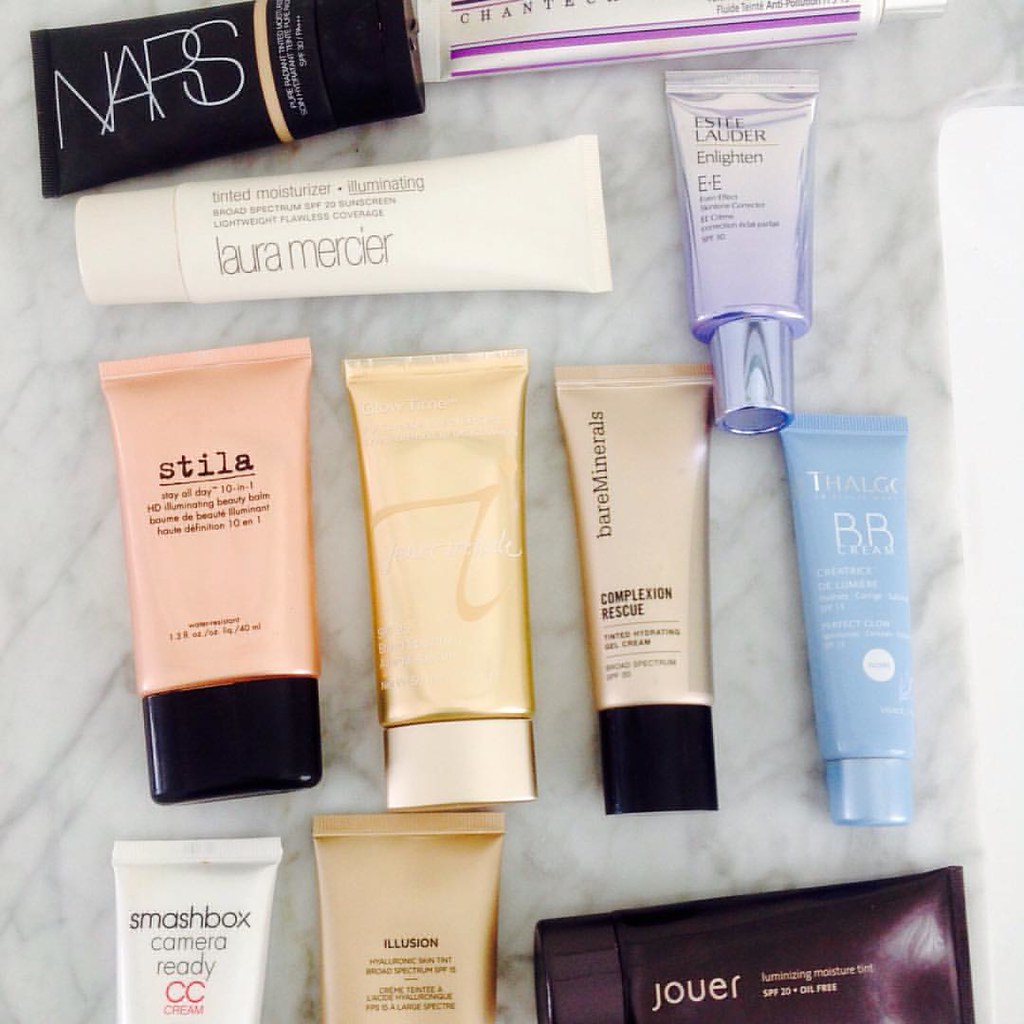The image showcases a diverse array of makeup products from a variety of brands, each with unique packaging and features. At the top, there are several NARS products encased in sleek black containers. These containers are designed to be unscrewed at the bottom, revealing a squeezy tube applicator. To the right of the NARS products, there is a white container adorned with purple stripes, though the brand information is not clearly visible.

Directly beneath the NARS items, a Laura Mercier product can be seen. It is a tinted moisturizer with illuminating properties, offering broad-spectrum sunscreen and promising lightweight, flawless coverage. Positioned to the right of this is the metallic purple Estee Lauder Enlightened EE Cream, which stands out with its lustrous finish.

On the row beneath these items are four vertically aligned products. First is the Stila Stay All Day 10-in-1 HD Illuminating Beauty Balm. To its right is a gold container with a reflective surface, making the brand name difficult to discern, though it appears to say "Glow Time." Following this, there is the Bare Minerals Complexion Rescue, a tinted moisturizer gel cream. Next to it, a smaller baby blue tube houses a BB cream from Falgeo.

In the bottom left corner of the image, only the tops of two containers are visible: the Smashbox Camera Ready CC Cream and a product labeled "Illusion Hyaluronic Something Tint Broad-Spectrum SPF." Finally, laying horizontally is a dark purple tube identified as Jouer Illuminating Moisture Tint. The assortment presents a rich variety of makeup essentials, each catering to different skincare and cosmetic needs.